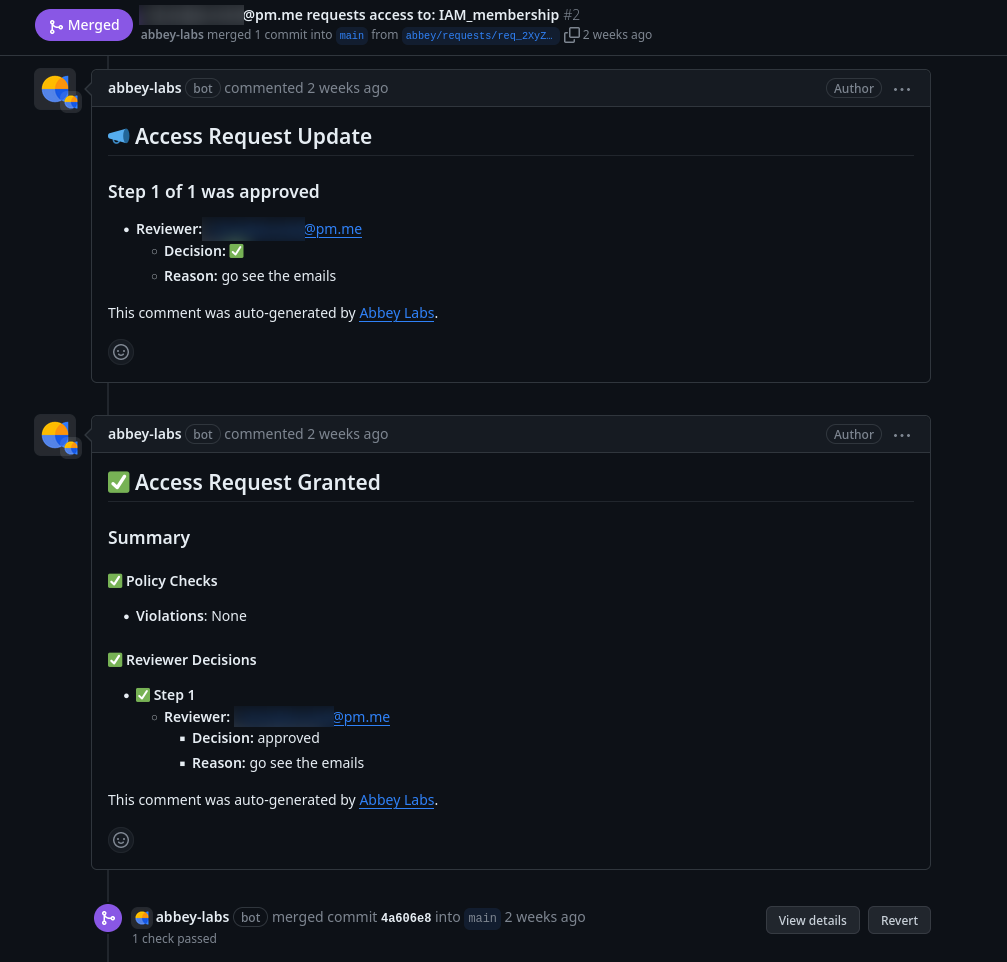This image displays a user interface element, likely from a version control or code collaboration platform. The primary focus is a purple 'Merge' button situated on the upper left side, shifted slightly to the right to indicate indentation. The background of the interface is predominantly black. Adjacent to the right of the 'Merge' button, there is a redacted section labeled "apppm.me" which suggests a web address or identifier that has been obscured. Below this, the text reads "Request access to im_membership_number_two."

Further down, we see a detailed activity log. It notes that a user named "abbylabs" merged one comment into the main branch from "abby/request/req_2xyz_," an action that took place two weeks ago. Below this entry, two additional sections are visible, each labeled with "abbylabs." These sections appear to be comments, both also timestamped from two weeks ago, indicating user interactions or feedback on the code or content in question.